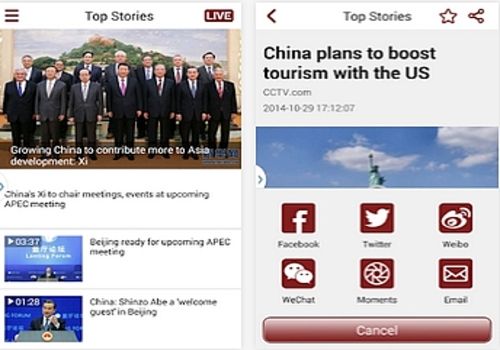This image depicts a low-quality screenshot of an older user interface from an unspecified app, seemingly updated but still retaining a dated design. The screenshot is divided into two sections, each showing different pages of the same app. 

On the left-hand section labeled "Top Stories," there's a "Live" indicator in the upper right corner, suggesting real-time updates. Prominently featured is a banner headline: "Growing China to Contribute More to Asia Development," along with a secondary subtitle stating, "China's Xi to Chair Meetings, Events at Upcoming APEC Meeting." 

Below the main banner, there's a smaller icon labeled "Videos," accompanied by several subtitles including, "Beijing Ready for Upcoming APEC Meeting," and "China, Shinzo Abe, a Welcome Guest in Beijing." These details date the screenshot, as Shinzo Abe, the former Japanese Prime Minister, was assassinated in 2022.

The right-hand section illustrates how users can share a top story. It features a headline that reads, "China Plans to Boost Tourism with the US," attributed to cctv.com and dated October 29, 2014, at approximately 5 PM. Sharing options are visible, including platforms like Facebook, Twitter, Weibo, WeChat, Moments, and email, indicating the app's release around that time.

The combination of timestamps, historical context, and sharing options offers insight into the specific era and functionality of this app interface.